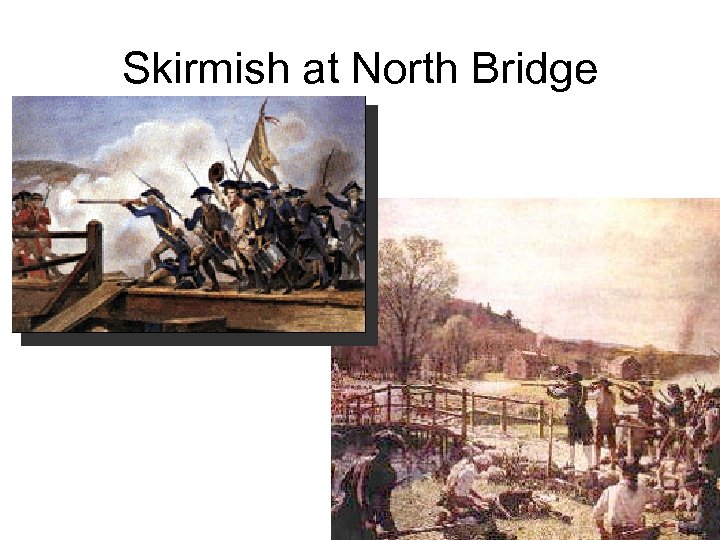The image, titled "Skirmish at North Bridge" in bold black font at the top, consists of two side-by-side illustrations against a white background. The illustration in the upper left corner depicts a battle scene from the Revolutionary War era. In this scene, colonial soldiers, identifiable by their attire, are engaged in combat on a pier or bridge. To the right, blue-coated soldiers hold up a flag amidst a backdrop of blue sky and a cloud of musket smoke. On the left, a couple of red-coated soldiers can be seen, suggesting a confrontation. The second illustration in the lower right corner features a muted, tan-colored depiction of a countryside skirmish. Here, militiamen equipped with muskets stand on the right side of a small wooden bridge. The background reveals rustic wooden cabins, trees, and distant mountains, enhancing the pastoral setting. In the foreground, some men are seated on what appears to be stumps, adding depth to the scene. The cohesive theme captures contrasting yet complementary scenes from the same historical conflict at North Bridge.